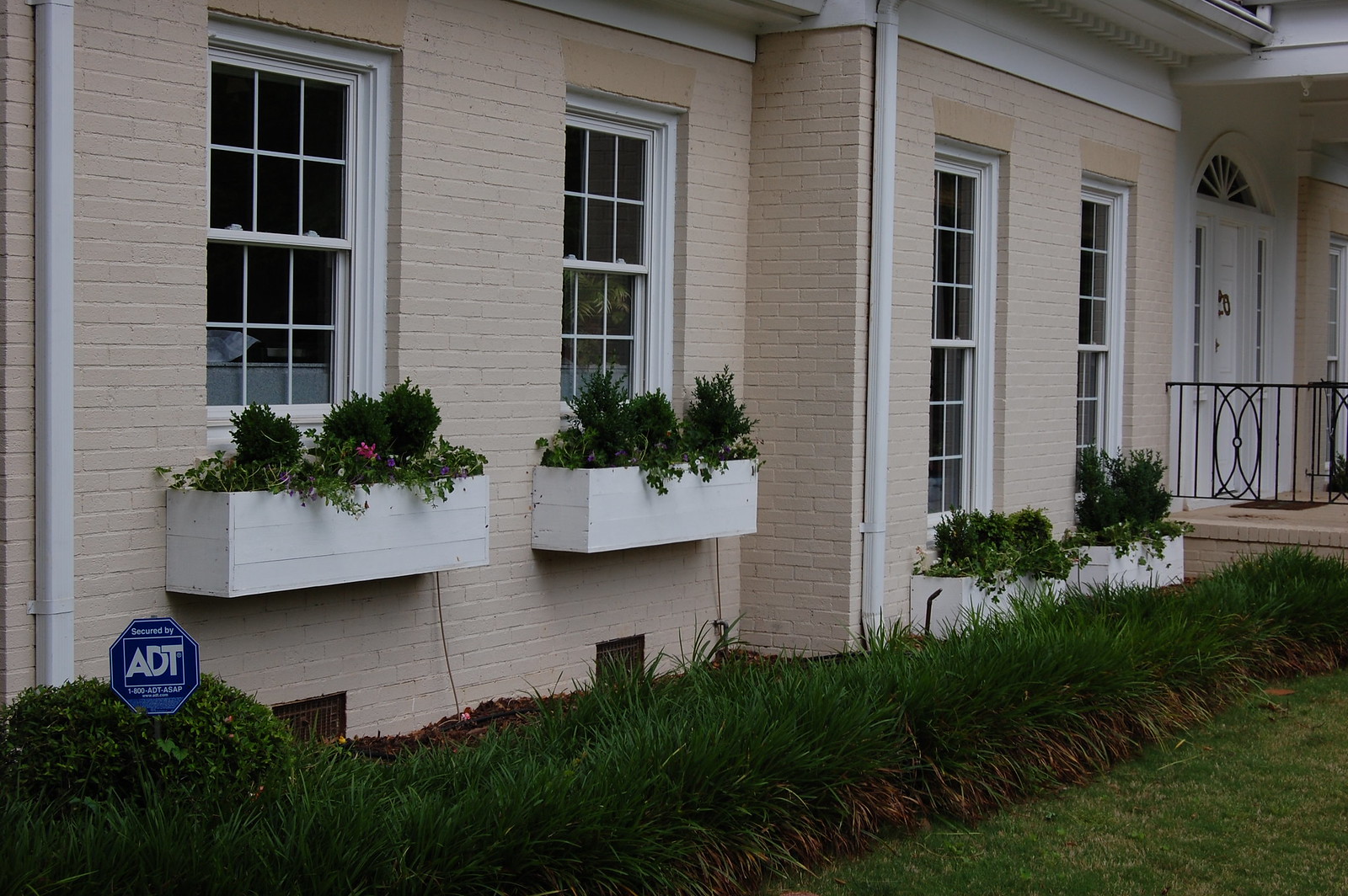This image captures a beautifully maintained, older brick mansion painted in a pale pinkish nude color. White accents adorn the house, including downspouts, window frames, flower boxes, and a large front door. The front door features an elegant half-circle transom window above it and is accessible via a small entry porch with a decorative, black wrought iron railing. Along the front of the house, carefully manicured green bushes line the base of the picture windows, which are interspersed with vibrant flower boxes containing green plants and small pink flowers. A lush, dark green lawn stretches out in front, enhancing the home's charming, timeless appeal.